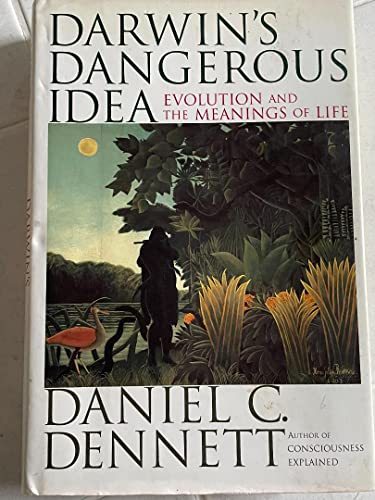This image depicts the cover of the book "Darwin's Dangerous Idea: Evolution and the Meanings of Life" by Daniel C. Dennett, author of "Consciousness Explained." The mostly white cover features an illustrative painting centrally placed on the front. The artwork depicts a silhouetted figure, possibly a hunter or a person playing a flute, standing beside a riverbank with tall grass and plants. Near the figure's feet is an orange or possibly duck-like bird, while in the background, a yellow moon or sun hovers above the horizon amidst some clouds. To the right of the silhouette, a dense forest with sprouting shoots can be seen, and the scene’s natural details suggest a jungle or thickly vegetated area. The painting is signed by the artist in the lower right corner, adding a personal touch to the serene yet evocative imagery.